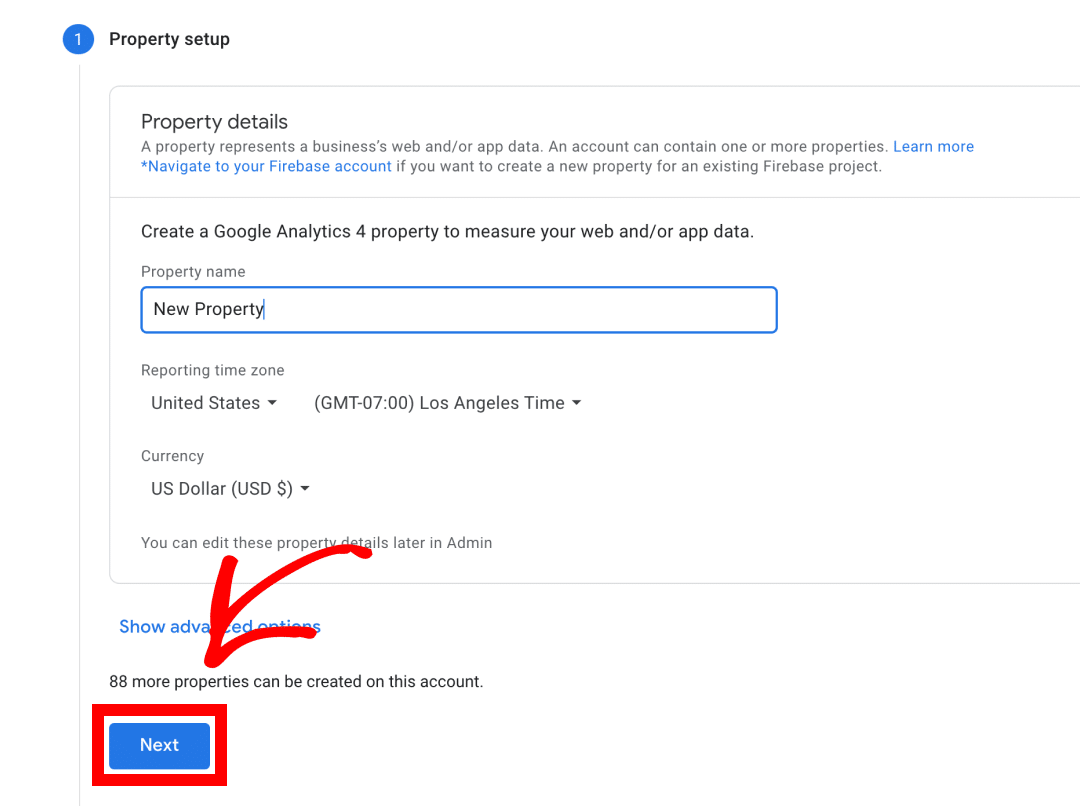The image showcases a "Property Setup" configuration screen for creating a Google Analytics 4 property. At the top, marked with a blue circle containing the number "1," the title "Property Setup" is prominently displayed. Directly beneath, within an information bar, the section titled "Property Details" includes the slogan: "A property represents a business's web and/or app data. An account can contain one or more properties. Learn more."

Further instructions advise users to "Navigate to your Firebase account if you want to create a new property for an existing Firebase project." Below this, the option to "Create Google Analytics 4 property to measure your web and/or app data" is presented.

In the form fields, someone has entered "New Property" for the property name, selected "United States, GMT-0700 (Los Angeles time)" as the reporting time zone, and chosen "US Dollar" as the currency.

To highlight the next step, the image has been digitally edited: a red box surrounds the "Next" button, and an arrow drawn in red paint points directly at it, indicating that the user should click this button to proceed to the following page or the next part of the setup process.